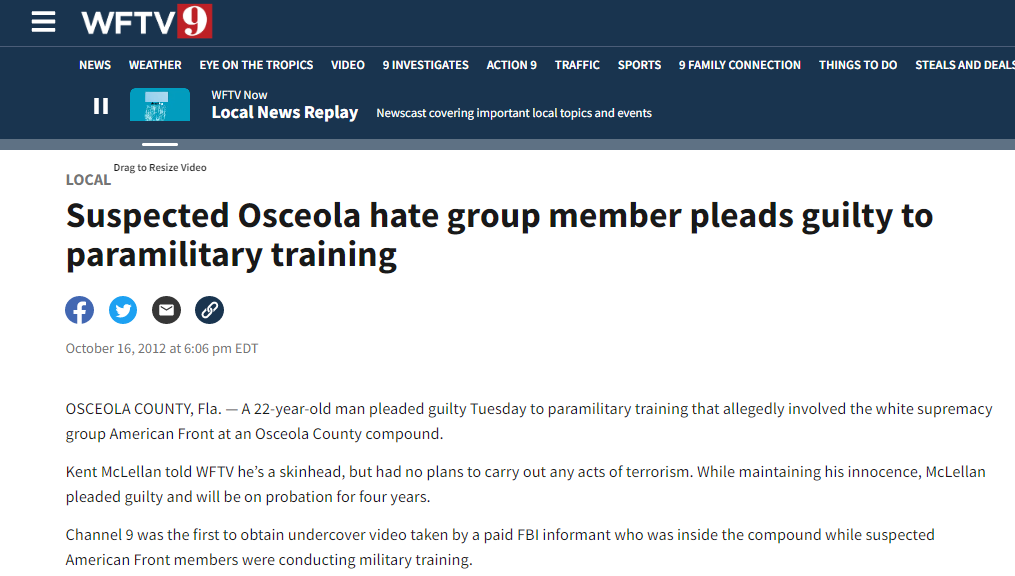The image features a black header at the top showcasing the WFTV logo, a red square with a white number nine inside it. Below the logo, a list of sections and features are displayed: "News," "Weather," "Eye on the Tropics," "Video," "Nine Investigates," "Action 9," "Traffic," "Sports," "Nine Family Connection," "Things to Do," "Steals and Deals," "WFTV Now," "Local News," "Replay," and "Newscasts Covering Important Local Topics and Events."

The main content conveys a news story headline: "Local Suspected Osceola Hate Group Member Pleaded Guilty to Paramilitary Training." Social media sharing icons are positioned underneath the headline.

The detailed news report follows:
Dated October 16, 2012, at 6:06 PM EDT in Osceola County, Florida, it describes a 22-year-old man's guilty plea on Tuesday concerning charges of paramilitary training alleged to involve the white supremacy group, American Front, at an Osceola County compound. The individual, Kent MacLellan, admitted to being a skinhead but denied any intentions of carrying out acts of terrorism while maintaining his overall innocence. Despite his claims, MacLellan's guilty plea results in a four-year probation sentence. Notably, WFTV Channel 9 was the first to secure undercover video related to the case.